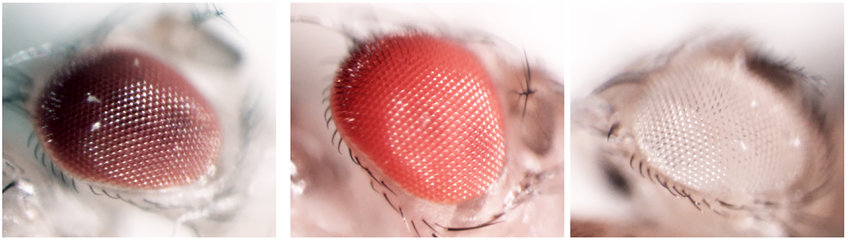In the image, we see a sequence of three panels displaying the same multi-faceted object, resembling an insect eye or mesh. The first panel features the object in a deep red color, set against a transparent or silver background. Surrounding the object are fine, hair-like structures that appear like eyelashes. The middle panel shows the object in a bright red hue with the same lash-like structures encircling it. The background in this panel is also light, possibly white. The final panel presents the object transformed to a silver or white color, still surrounded by the eyelash-like structures. The background here transitions to a light pink shade. All three images are positioned side by side, depicting an evolution in color while maintaining the same intricate, multi-faceted texture and surrounding details. The overall setting suggests an indoor photoshoot, with a bird's-eye view of the objects.